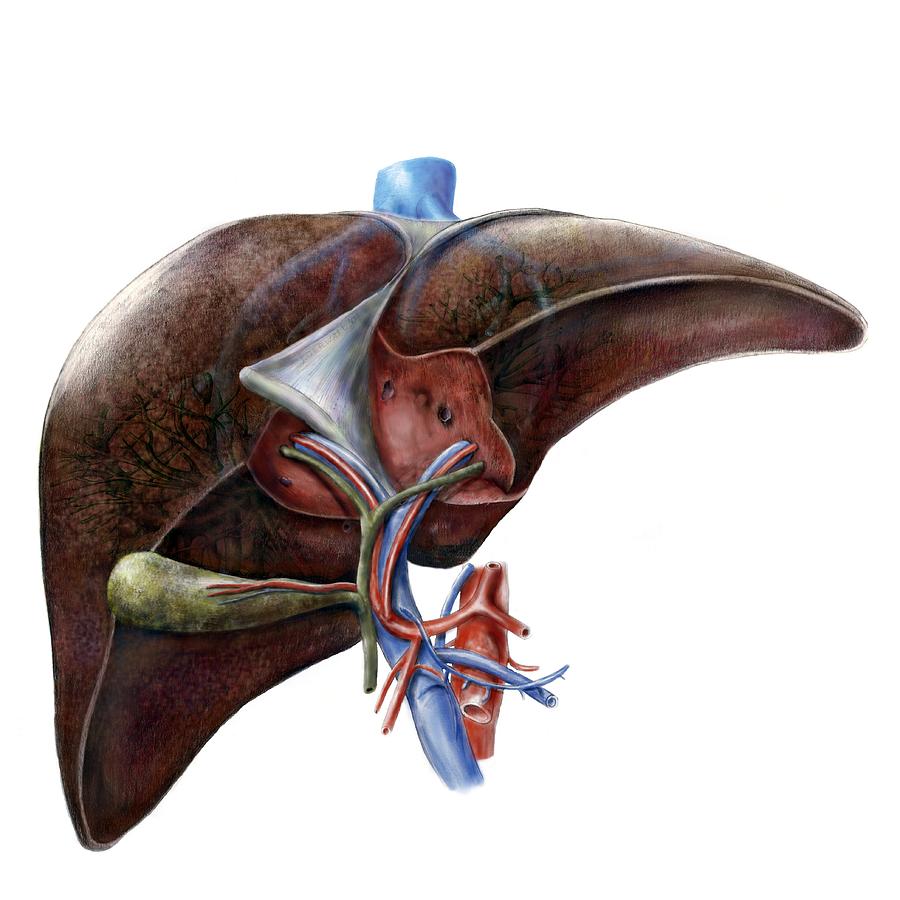The image is a high-quality illustration of a human liver, showcasing its anatomical details with great precision. The liver is depicted in a dark brownish-red color, suggesting its natural appearance. Prominently featured in the illustration are the primary blood vessels, with the arteries highlighted in red and the veins in blue, signifying the inflow and outflow of blood. The vessels can be seen branching off and penetrating the liver, illustrating the portal circulation. Additionally, a greenish gallbladder is attached to the liver via bile ducts. The liver has a smooth edge at the bottom, with a curved top that is concave. The intricate network of smaller blood vessels within the liver is also visible, emphasizing the organ’s complex vascular structure. This detailed diagram serves as an excellent educational tool for understanding liver anatomy and blood flow.